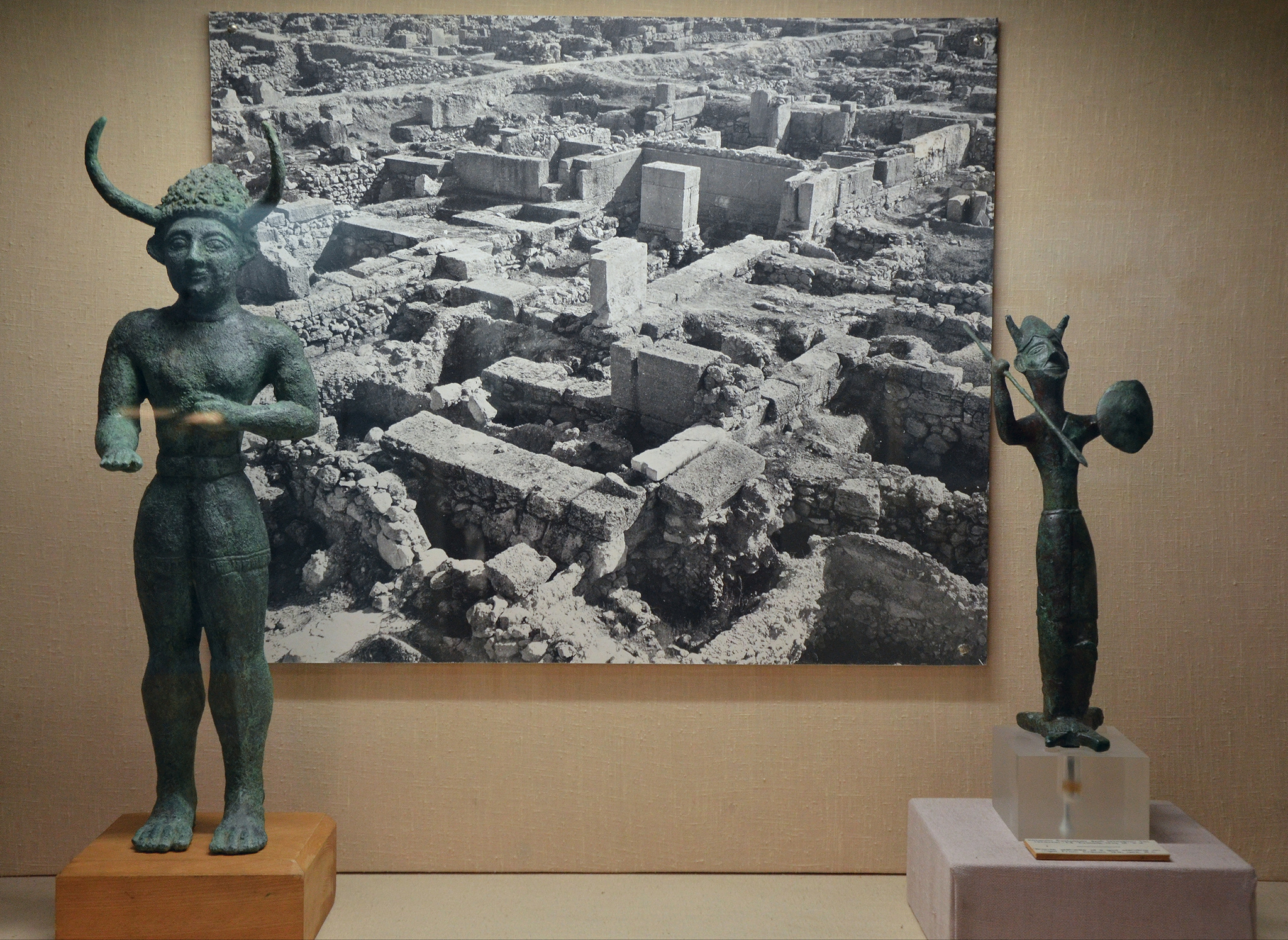The image depicts the interior of a museum showcasing historical artifacts and ancient relics. Central to the exhibit is a large, monochromatic photograph representing the ruins of an excavation site, marked by scattered stone blocks on the ground, evoking an ancient civilization. On the left side of the image stands a statue of a barefoot man in a green patinated hue, indicating it was likely made from copper that has oxidized over time. The statue features a helmet adorned with horns and extends its right arm. It is mounted on a brown pedestal. To the right, there is a smaller statue of a thin warrior figure, also displaying a helmet with horns and holding a spear. This statue stands on a glass-like pedestal. The overall color palette of the scene includes various shades of gray and white, contributing to the antiquated feel of the exhibit.